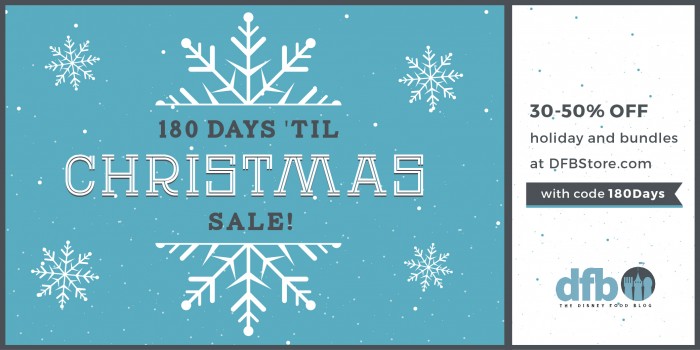The image portrays a promotional webpage with a distinctive color scheme divided vertically. The left side features a rich blue background adorned with four snowflake-like motifs: one at the top, one at the bottom, and two more on the left and right sides. Centrally positioned on this blue side is a large, bisected snowflake with one half extending upwards and the other downwards, splitting a series of promotional text.

The central text starts in bold black with "180 DAYS 'TIL" followed by "CHRISTMAS" in a mid-gray shade. Below this, "SALE!" is prominently displayed in bold black.

On the right side, the background shifts to white with small specks of dark blue scattered at the top and bottom. Centrally placed is an announcement in black text reading "30-50% OFF," followed by "HOLIDAY" and "BUNDLES" at DFB-Store.com, both in bold. A black rectangle further divides the section, containing white text: "WITH CODE," and in bold, "180 DAYS."

At the bottom, "DFB" is written in cyan blue, accompanied by a logo featuring three symbols within a circle: a fork-like object, a building-like structure, and a round shape.